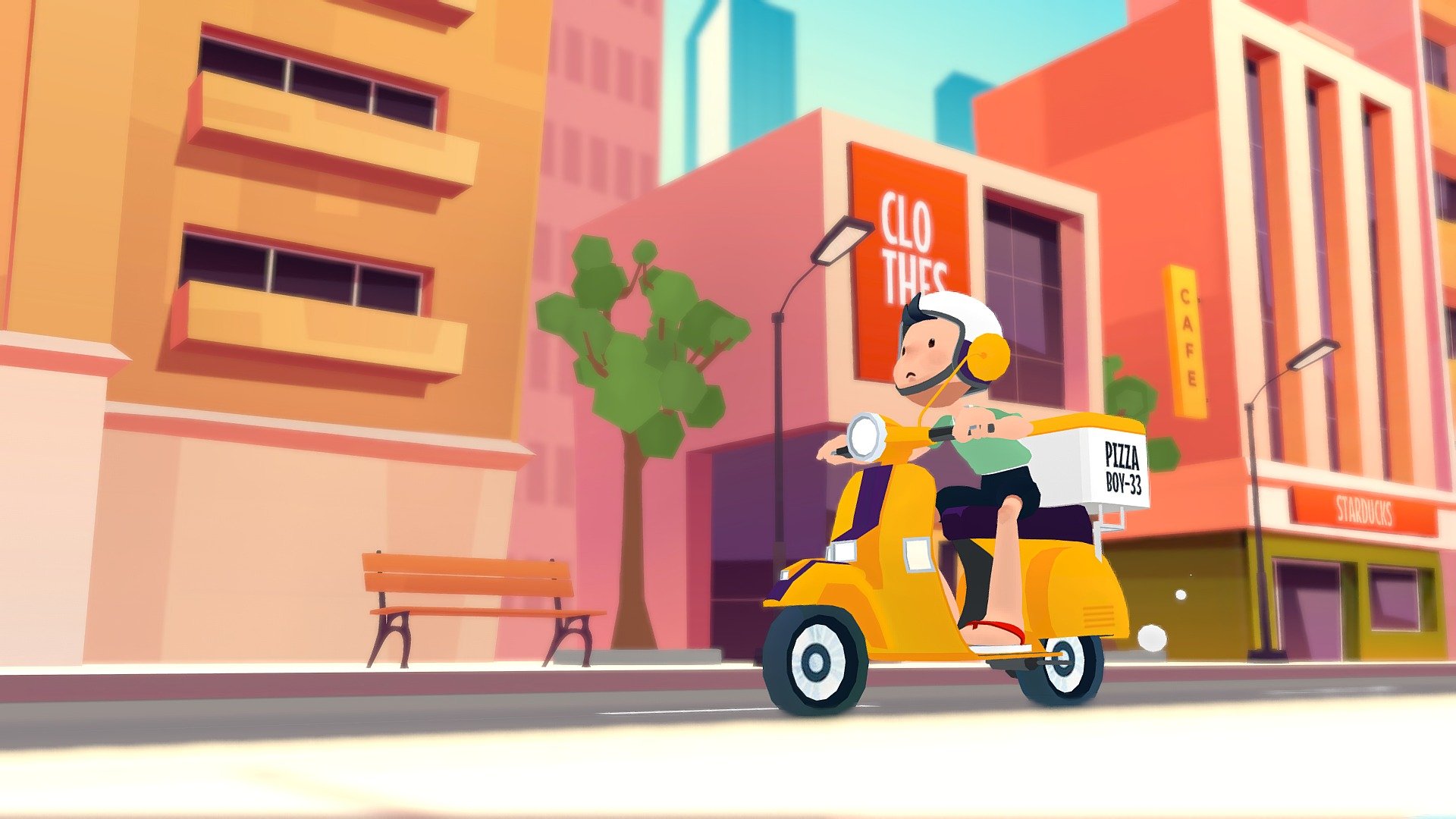The image is a vibrant digital illustration, likely a screenshot from a TV show or cartoon, depicting a bustling city scene. At the center, a boy in a green shirt, shorts, and flip-flops is riding a yellow moped with a purple stripe, delivering pizza as indicated by the "PIZZA BOY 33" written on the white delivery box attached to the back. He wears a white helmet with a yellow circle on it, conveying a look of concern, possibly because he’s lost or in a hurry. The cityscape in the background is colorful and simplified, featuring tall skyscrapers, various buildings like an orange one with a pink base, a pink building labeled 'clothes,' and another building that resembles a closed café named 'Star Ducks.' There's also a bench, a tree with green leaves, and a street light enhancing the urban setting. The bright and sunny atmosphere, along with the detailed yet cartoonish style of the illustration, brings the dynamic city scene to life.